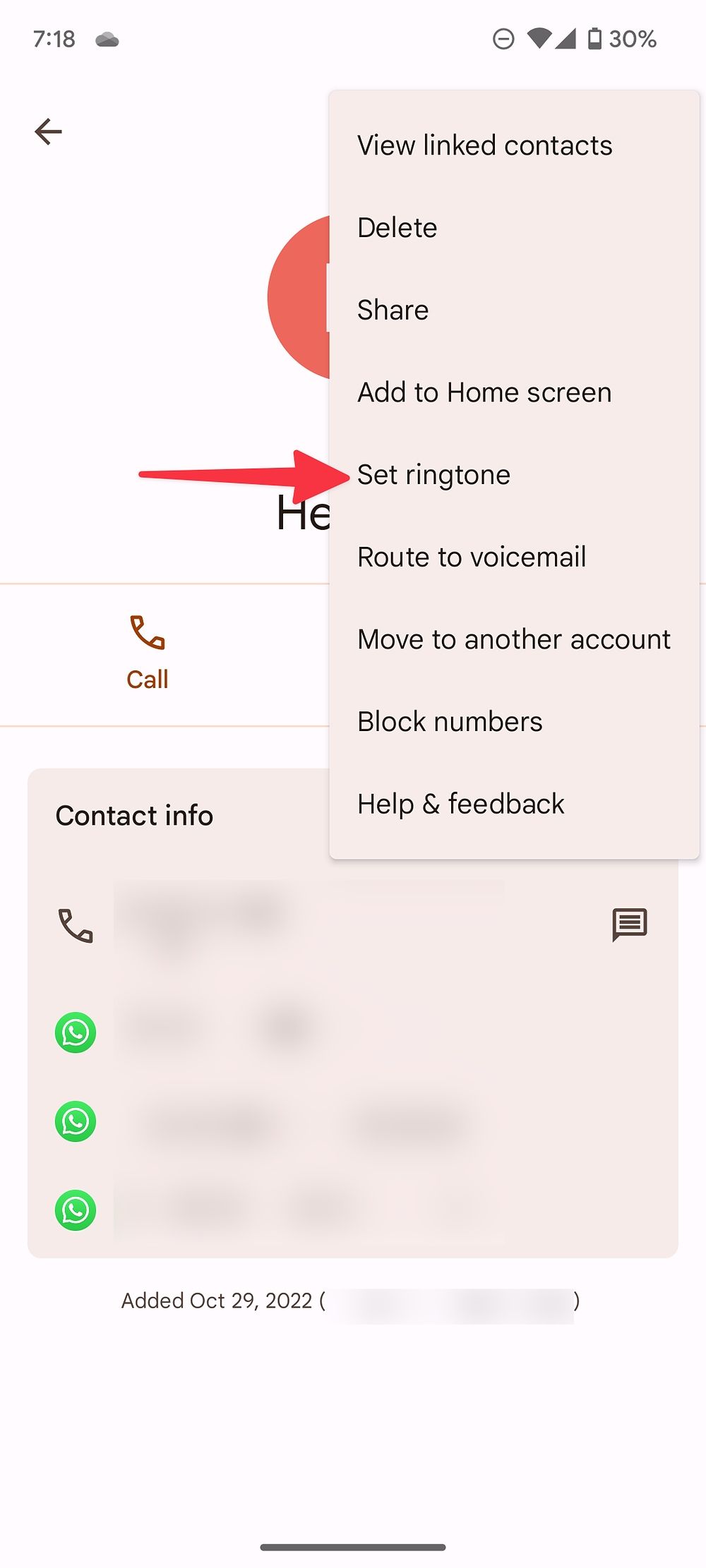This screenshot from a mobile phone displays the settings menu within the call app. The image, taken at 7:18, reveals a battery level of 30% in the upper right corner. The background is predominantly white. Central to the screenshot is a red arrow highlighting the "Set Ringtone" option within the app's menu. 

In the bottom section of the screenshot is a blurred area labeled "Contact Info," concealing the private details of the individual for whom the settings are being configured. Below this, a simple pencil-drawn phone icon is visible, followed by three additional phone icons encased in green circles.

Positioned centrally within the app is a call button, which allows users to initiate a call to the contact whose details are on display. The page also notes that this contact was added on October 29, 2022.